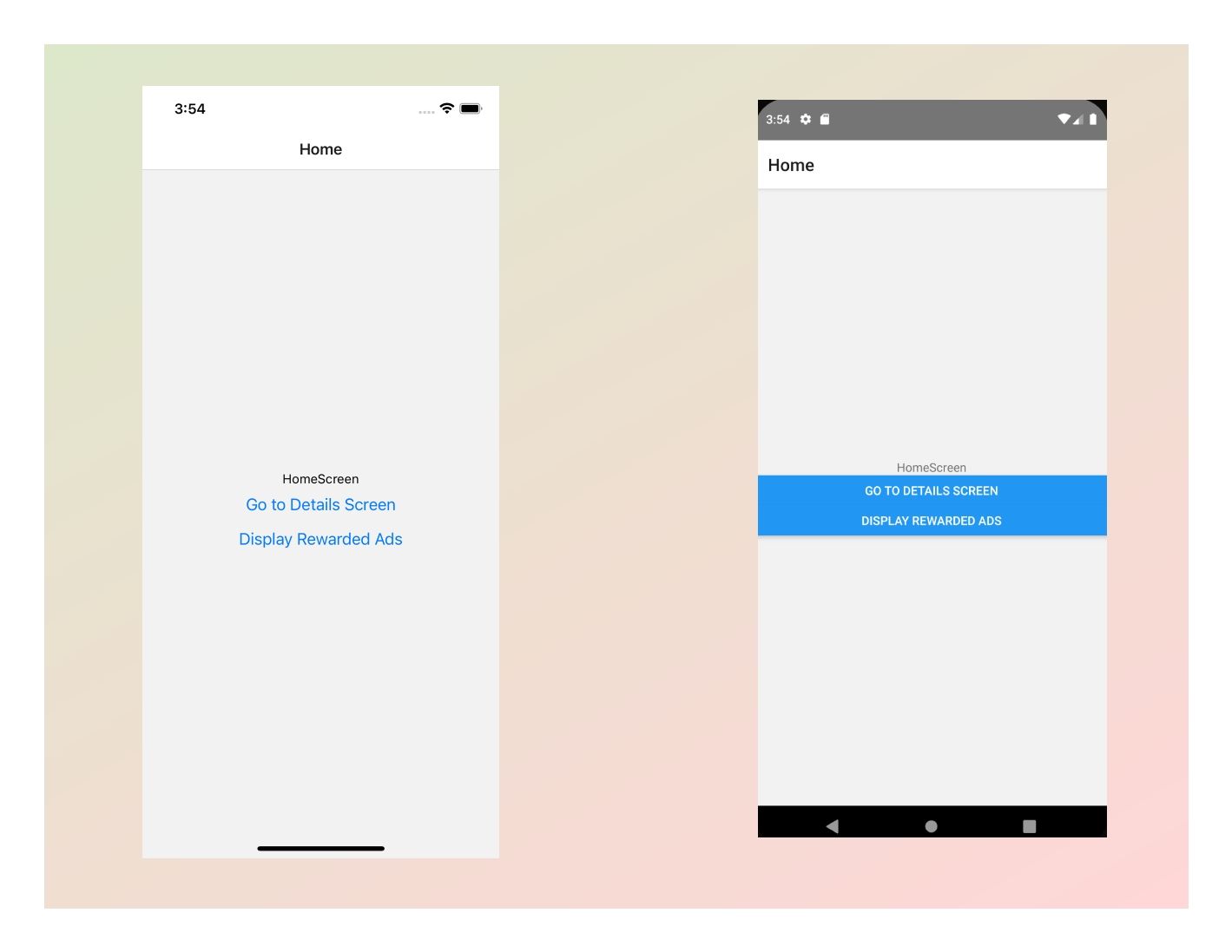In the image, there is a blush-pink/nude colored background, giving it a soft, subtle atmosphere. The image appears to be an edited composition containing two separate screenshots, presumably taken from two different cell phones. 

**Left Screenshot:**
The background of the screenshot is predominantly white. At the very top, the status bar displays the time "3:54," the WiFi signal icon, and the Birchie application logo, all in black text/icons against the white background. Below the status bar, a grey section contains the word "Home" in black ink. Further down, the screen conveys black text indicating various options, including "Home Screen," "Go to Detail Screen" in blue ink, and "Display Rewired Ads" also in blue ink.

**Right Screenshot:**
This screenshot features a darker theme with a black background partially obscured by a grey strip at the top displaying the same time, "3:54," along with icons for settings, memory card, battery percentage, and WiFi. Below this grey strip, a white background is present with the word "Home" written in black ink. The grey background continues below with the words "Home Screen" in grey ink. Additionally, the options "Go to Detail Screen" and "Display Rewired Ads" appear in the text box with white text on a blue background.

The consolidated visual of these two screenshots over the pink/nude backdrop creates an intriguing yet detailed composite image.